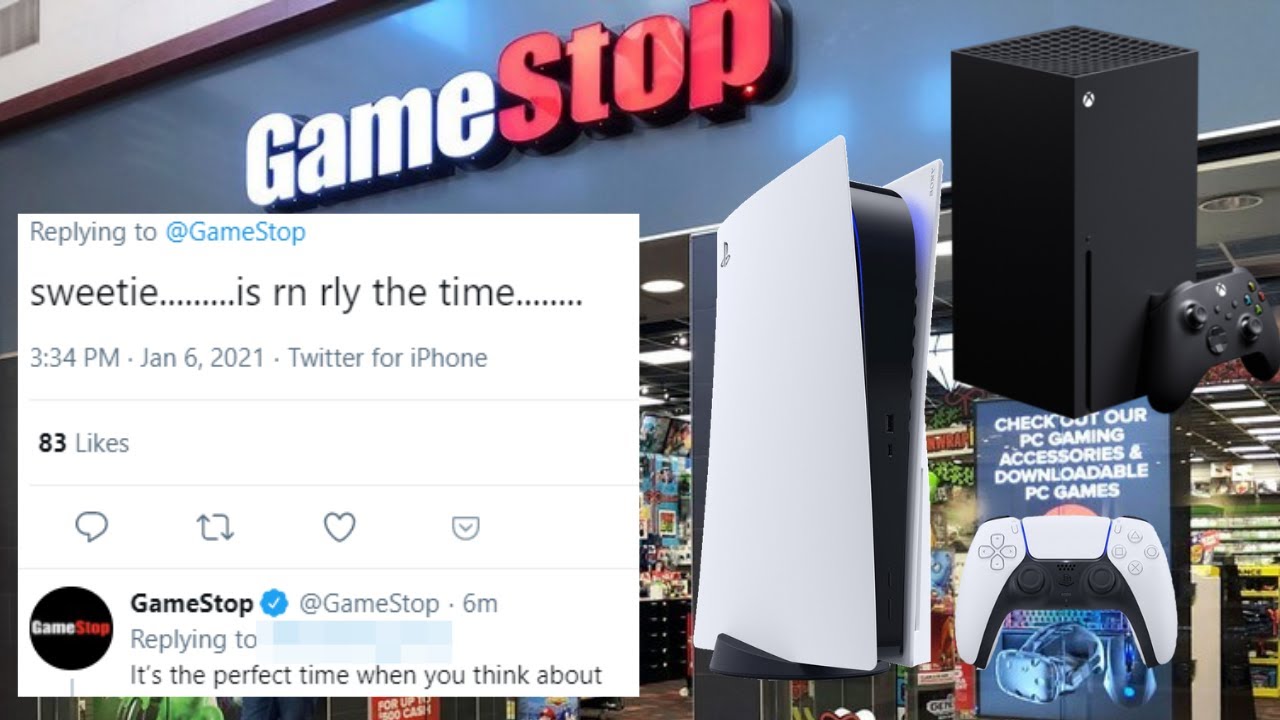The image captures the interior of a mall, prominently featuring a GameStop store. The store's entrance displays the recognizable GameStop logo, with "Game" in white and "Stop" in red set against a dark blue background. However, the view into the store is somewhat obstructed by a suspended speaker, mounted in the air, which somewhat resembles a TV mount. Additionally, a Game Boy or similar console is visible, further limiting the clear view of the store's interior.

Overlaying the image, a Twitter notification is evident. It shows a tweet from a user replying to GameStop, marked with the handle and timestamp: “Sweetie, @3:34 PM · Jan 6, 2021 · Twitter for iPhone.” The tweet text appears to reference the perfect timing of the event, but it ends abruptly, leaving the full context unclear.